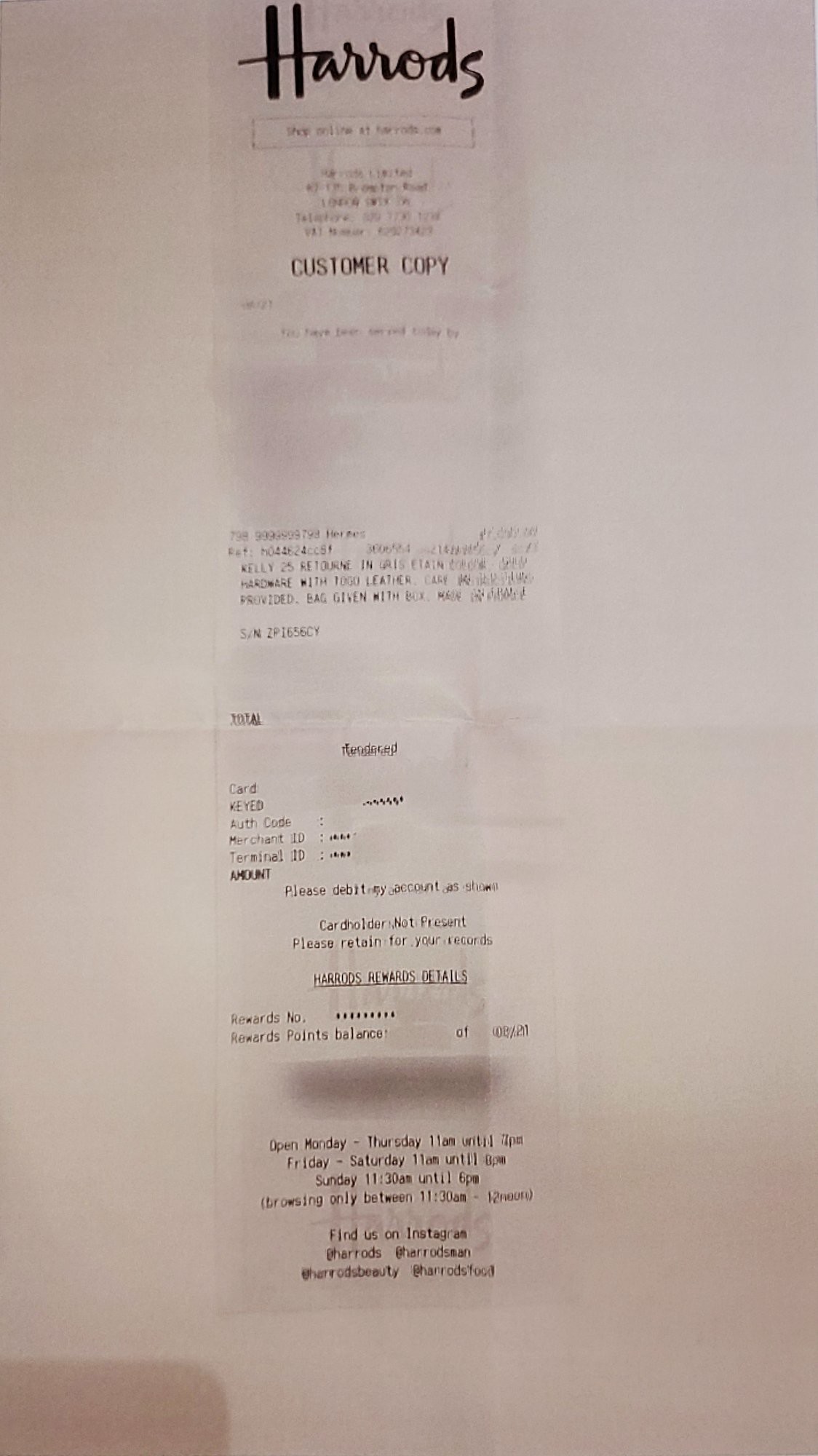This image captures a scanned receipt placed on a white sheet of paper, focusing on the detailed presentation of the receipt. At the top of the receipt, the word "Harrods" is prominently displayed in bold black letters, immediately signaling the store of origin. Underneath the store name, in smaller text, the label "Customer Copy" is clearly visible. The middle section of the receipt appears blurred, obscuring the specific items purchased and their individual prices. Both the total amount and the credit card information at the bottom of the receipt are also blurred for privacy, ensuring no sensitive data is visible. In the bottom left corner of the photo, there is a shadow cast by the edge of a cell phone, which partially intrudes into the frame, adding an element of context to the capture.